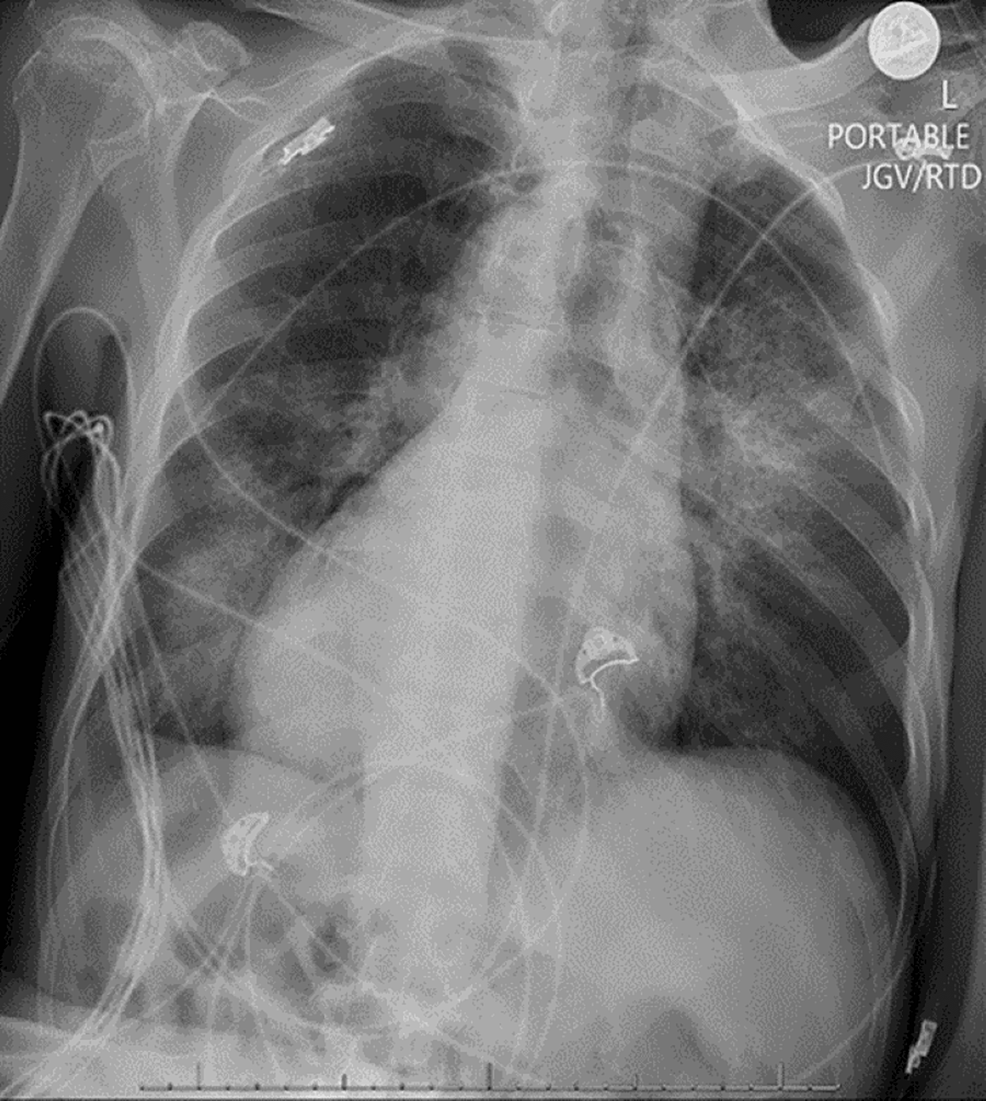This image is a black and white x-ray of a person's upper torso, primarily displaying the ribcage, shoulders, collarbone, and spinal cord. In the top right corner, there's text that reads "L Portable JGV / RTD." The ribcage and shoulder bones are clearly visible, while the arm bones are partially shown. Notably, there are two peculiar, dense shapes in the x-ray: one located centrally in the chest and the other in the lower left area of the torso. These shapes resemble small devices or implants and stand out against the otherwise identifiable ribs, spine, and organs. The unusual shapes have an almost organic appearance, described variably as resembling mushroom caps or jellyfish, and seem to be the focal point of the x-ray examination. The overall image is somewhat surreal, with these mysterious objects contrasting against the structured anatomy of the torso.